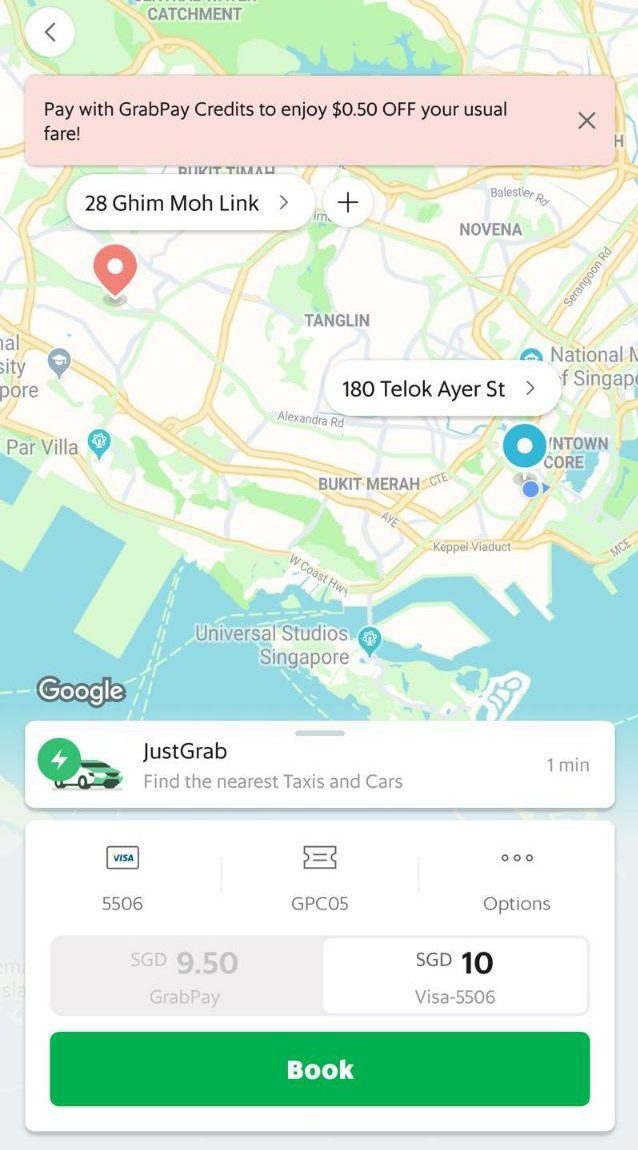Here is a cleaned-up and detailed descriptive caption for the given image:

---

The image depicts a smartphone screen showcasing a map of Singapore on a ride-hailing app. A promotional message at the top of the screen reads, "Pay with GrabPay credits to enjoy 50% or 50 cents off your usual fare." In the upper-left section of the map, there's a prominent pin location marked with the address "26 Jem Mo Link" or "28 Jem Mo Link," and another location "180 Telok Ayer Street" is also indicated.

On the map's interface, various navigational and functional icons are visible. The bottom section features labels from Google Maps, emphasizing the service's integration with the app. Just below the map, the app offers options to "Find the nearest taxis and cars" with an icon of a circle containing a lightning bolt and the text "1 minute," likely indicating the estimated arrival time of the nearest taxi or car.

The payment section displays options to pay with Visa, alongside a code labeled "GPC05." An "Options" button is also present, providing users with further customization and selection choices. At the very bottom, the payment methods "GrabPay" and "Visa" are shown, with Visa being selected. Adjacent to the payment options, a green "Book" button is prominently displayed, ready for the user to confirm their ride-hailing request.

---